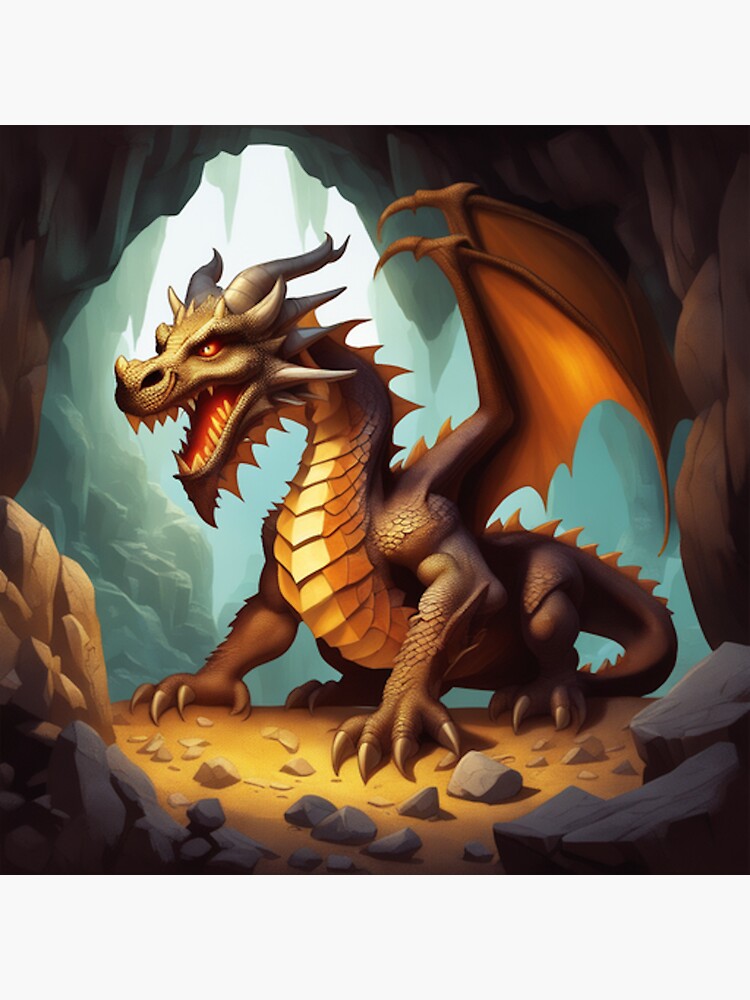The image depicts a detailed colored art illustration of a dragon in a cavern setting. The dragon, rendered in a 3D animation style, stands with its massive bat-like wings partially spread, their orange hues accentuated by spikes along the top. Its body is primarily a brownish-red color, with yellow-orange scales running down its chest and long, menacing brown talons on its feet. The dragon's head, turned slightly to the left, features a large, snarling snout filled with sharp teeth, glowing red eyes, and numerous spikes. Two prominent horns jut out from the top of its head among several smaller ones. The dragon's long, jagged tail bristles with orange spikes. The cavern setting is rocky with the ground colored in an orangish tone, and the dragon is dramatically silhouetted by bright white light streaming in from the entrance of the cave, casting shadows of blues and greens throughout the rocky interior. The overall atmosphere suggests the dragon's lair, bathed in an eerie, otherworldly light.